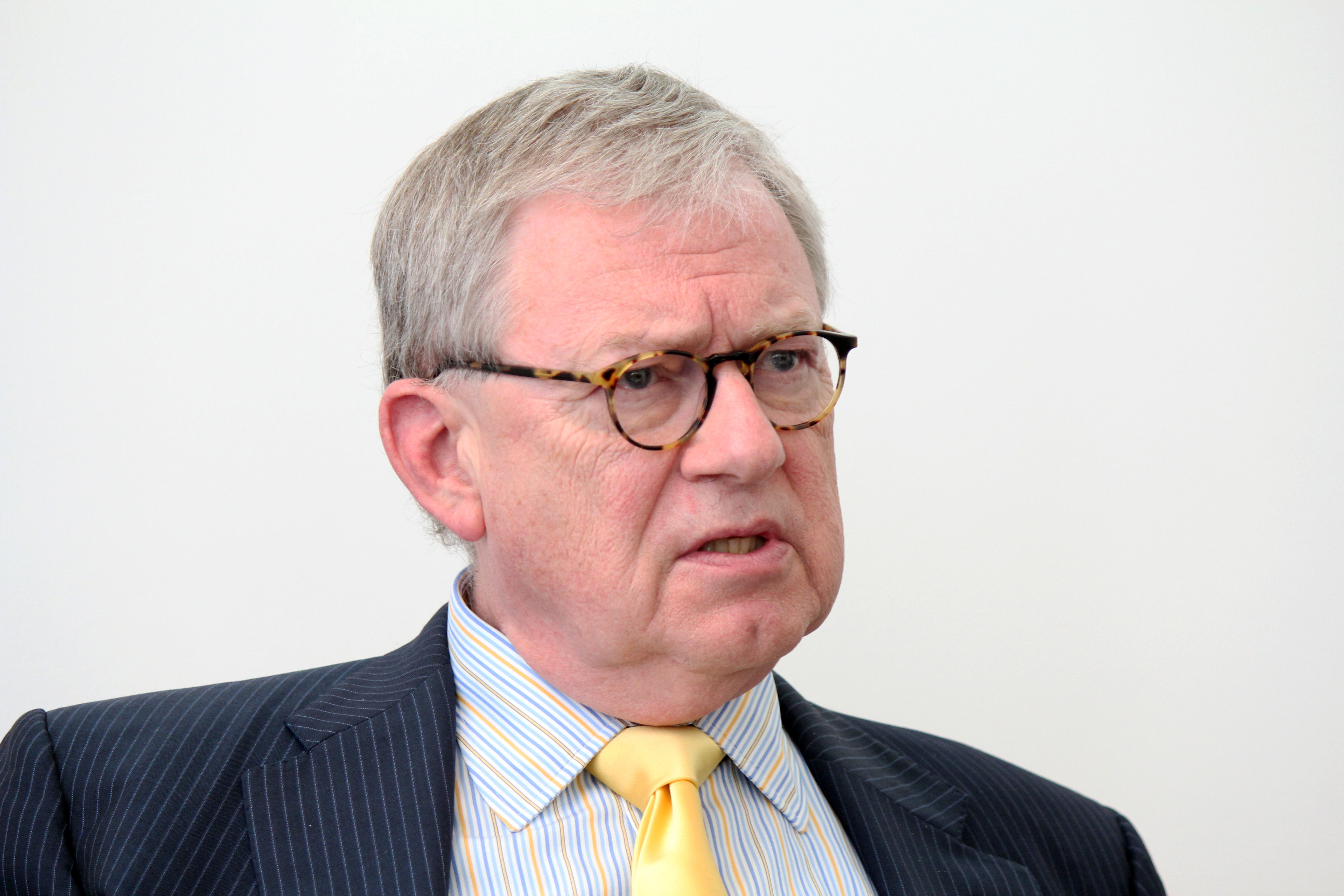The photograph features an older politician or spokesman, depicted from the shoulders up against a plain, white background. He has short, styled gray-white hair parted to the side, with facial expressions suggesting concern—his mouth slightly agape and eyes looking intently to the right. His face shows signs of age, with distinctive lines, wrinkles, and a characteristic dot in the middle of his chin. He wears round eyeglasses fitted tightly around his temples. His attire includes a dark blue pinstripe suit jacket over a multicolored shirt with intricate patterns incorporating pink, blue, dark, and light blue stripes, topped with a golden tie. The lighting, which is well-balanced, adds clarity to the details of his appearance, although it’s unclear whether it’s natural or artificial.